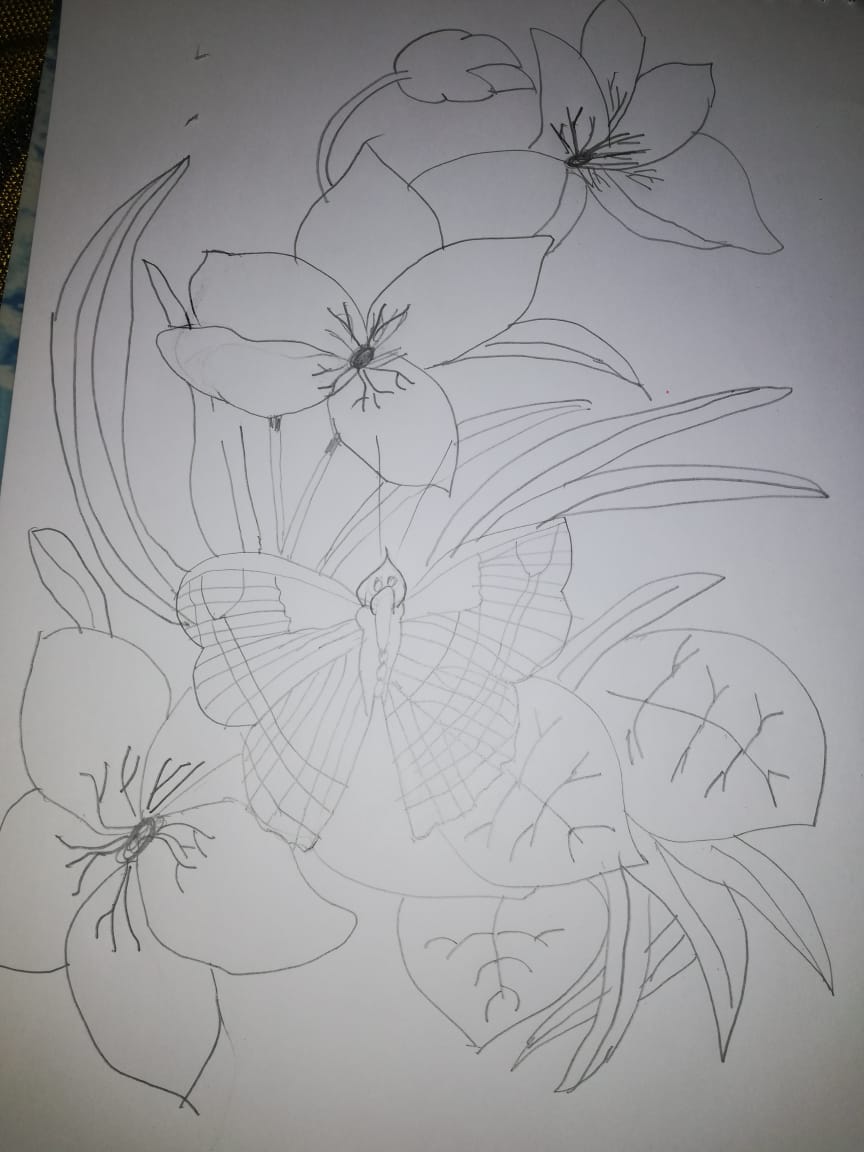This photograph showcases a simple yet detailed black and white line drawing created with a regular pencil on white paper. The centerpiece of the drawing is a butterfly adorned with several lines and designs on its wings, although the exact type of butterfly is not identified. Surrounding the butterfly are meticulously drawn tiger lilies, each displaying five distinct petals and visible pistils. There are also additional floral elements including a flower on the bottom left with visible petals, a group of three rounded-point leaves on the bottom right, and four narrow leaves that fan out. Above the butterfly, two flower blooms with five petals each are depicted, one situated slightly behind the other. Long blades of grass are sketched beneath the blooms, adding to the composition. The drawing features only outlines without shading or color, emphasizing the simplicity and elegance of the design. The surrounding elements outside the drawing in the photograph are minimal, possibly indicating some fabric to the left.